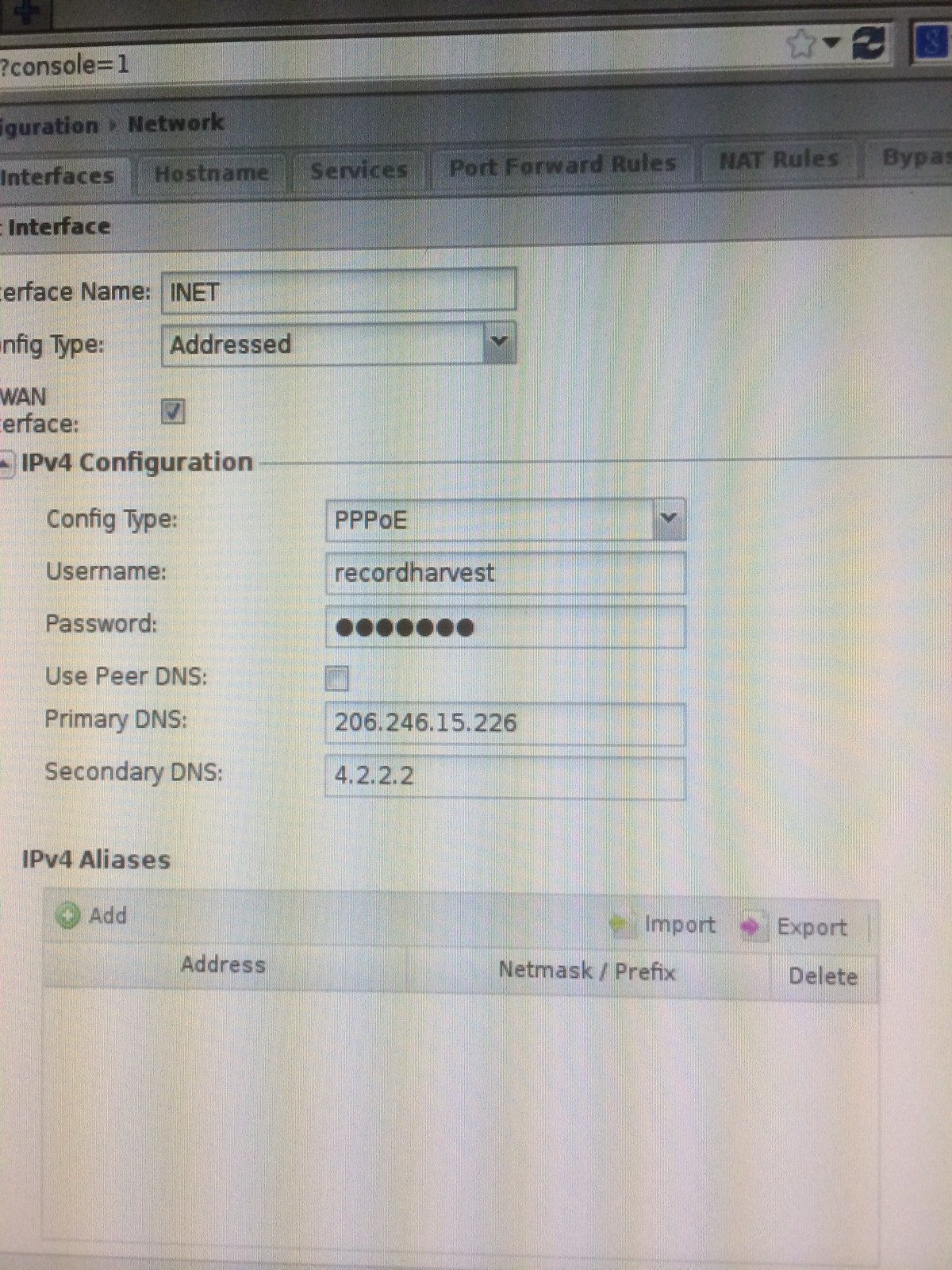The image captures a computer screen displaying a network configuration interface, taken with a camera that introduced lighting ripple effects typical of photographing screens. The interface tab is open, showing several menu options including Interfaces, Hostname, Services, Port Forward Rules, NAT Rules, and Bypass. The screen specifically delves into the details of the 'Interfaces' section under IPv4 configuration settings. Here, the interface name is listed as "inet" and the configuration type is "pppoe", with the username "recordharvest". The password is obscured, and the option to use peer DNS is unchecked. The primary DNS server is set to 206.246.15.226, while the secondary DNS is 4.2.2.2. The screen partially displays the address bar, indicating the query parameter "console=1". Additional network configuration details like IPv4 aliases, import and export address, netmask, and prefix options are also visible, providing a comprehensive view of the network setup.